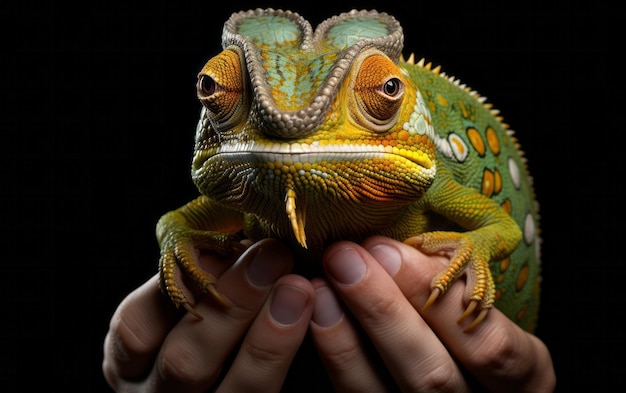The photograph features a strikingly detailed, vividly colored lizard, held carefully by two Caucasian hands against a stark black background. The reptile, primarily green, is characterized by an intricate pattern of orange and yellow hues, particularly around its eyes, forming a circular motif. A pronounced ridge starts from its nose, extending above its eyes into two rounded structures atop its head, adorned with a captivating blend of light blue and orange. Its thin, wide mouth is highlighted with white in the middle and yellow at the tips. The creature's legs exhibit a mix of orange and green, complementing the orange dots scattered along its green body. Sharp claws grip the person's fingers, while white spikes trail down its back and chin, adding to its exotic appearance. The lizard's eyes fixate directly on the camera, creating a sense of connection with the viewer, and its composed demeanor suggests a moment of calmness.